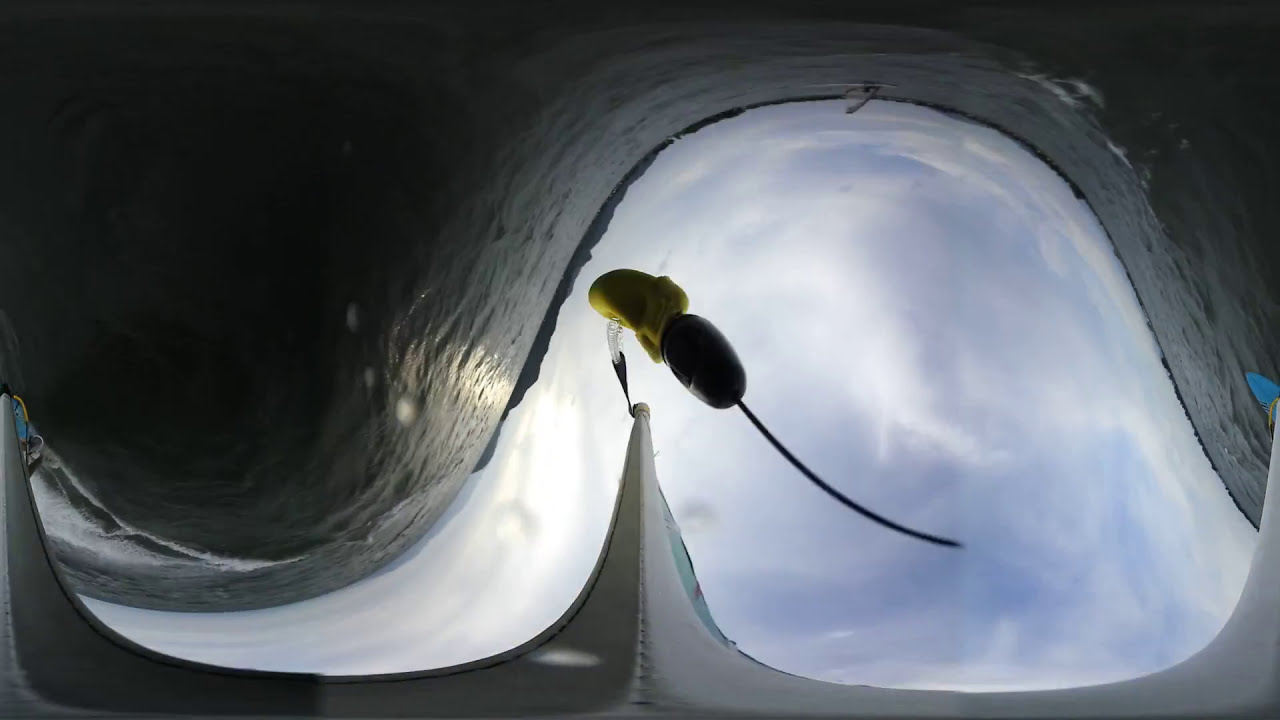The image is a highly distorted, fisheye or 360-degree photograph that makes everything appear curvy and surreal. At the center of the composition, there is a peculiar object with a long black tail at the back, and two oval shapes in the front, which might resemble sunglasses. The image features a prominent S-shaped curve that ascends and then descends, enclosing a light blue sky with scattered white clouds, creating the impression of looking up at the sky. This gives a disorienting effect as if the camera is mounted on a pole, possibly held by someone submerged in water. The photograph is further complicated by surrounding dark, almost blackish-green forms, possibly representing an ocean. Elements within the image hint at being partially blocked or obscured, with most areas being gray or black, contributing to the overall surreal and dreamlike quality.